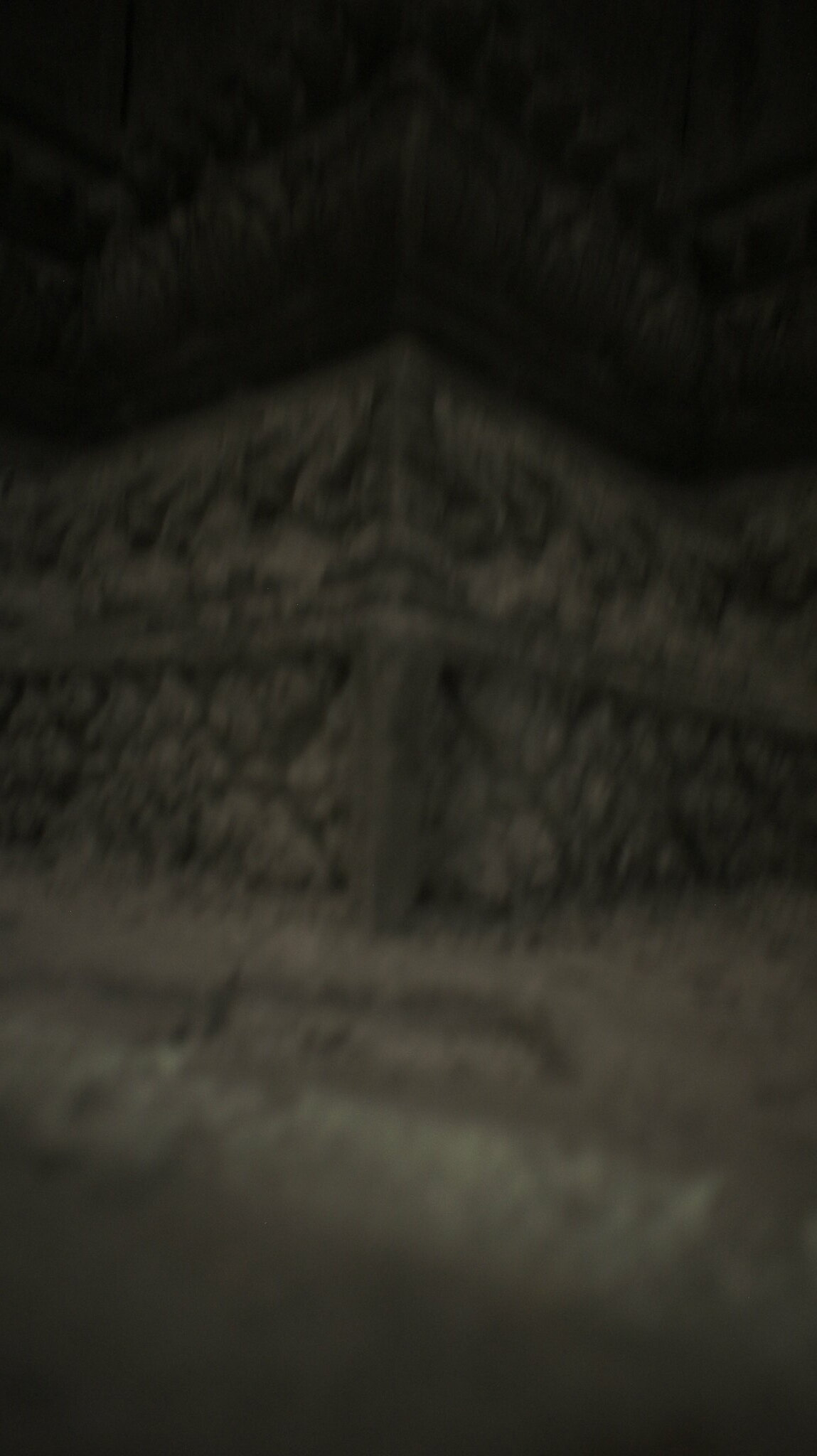The image is of notably poor quality, with a very low resolution and an overall blurry, fuzzy appearance, making it difficult to discern specific details. Predominantly indistinct, the image features a central surface or structure that extends in both horizontal directions, showcasing shades of gray and light gray. This structure appears to have some kind of design adorning it, though the details are obscure. Notably, towards the bottom portion of the structure, there are discernible diamond patterns, with a prominent circle situated at the center.